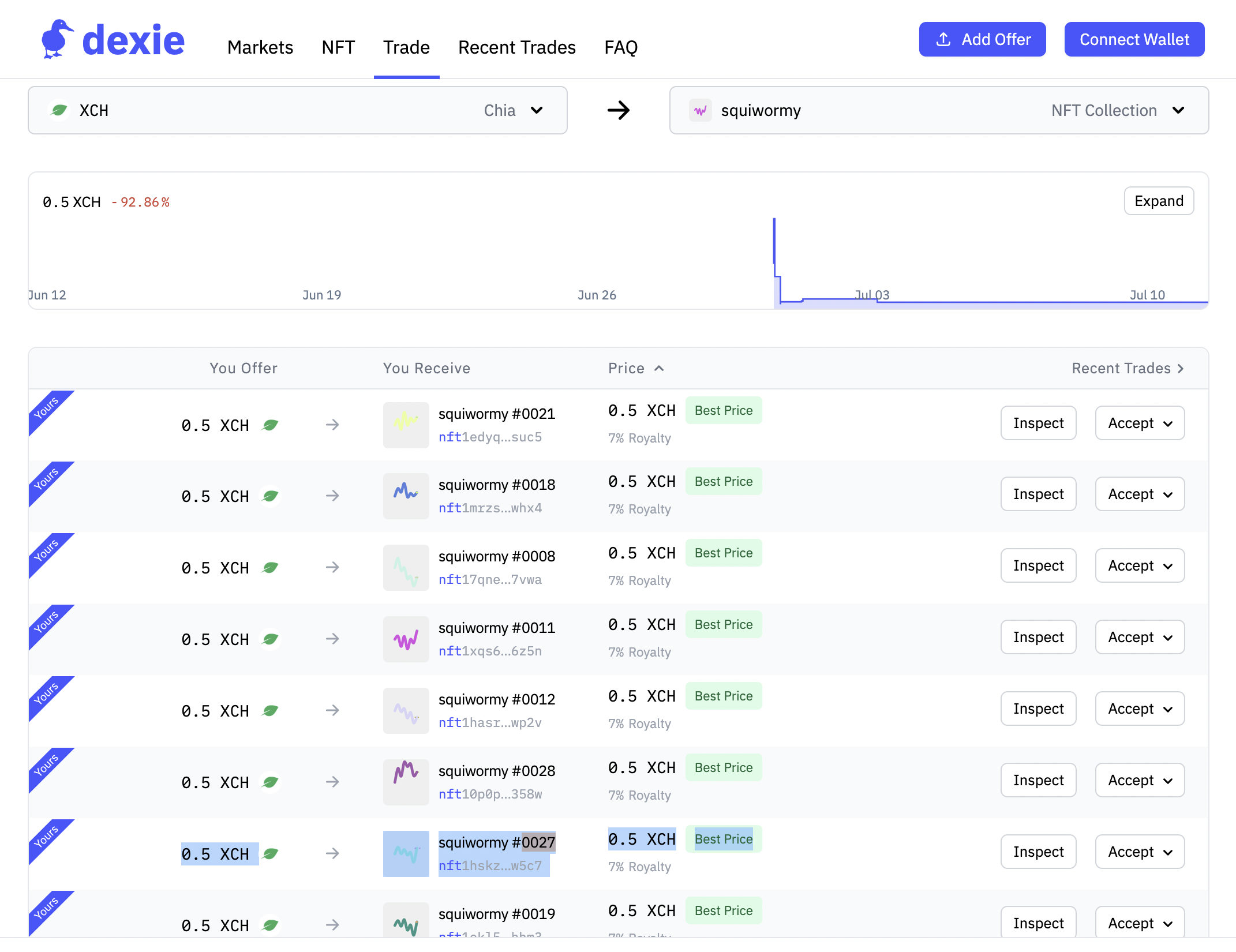The image appears to be a screenshot from a website featuring a blue duck logo in the top-left corner, labeled "Dexi." Adjacent to the logo, the navigation menu displays options including "Markets," "NFT," "Trade," "Recent Trades," and "FAQ," all in black text. Below the menu, two prominent blue buttons with white text are situated: "Add Offer" on the left and "Connect Wallet" on the right.

Further down, the interface features two search bars. The left search bar, marked with a green leaf icon, is labeled "XCH," while the right search bar is labeled "S-Q-U-I-W-O-R-M-Y" in black text.

Beneath the search bars, a grid of nine rows displays different objects. Each row lists "0.5 XCH" followed by "S-Q-U-I-W-O-R-M-Y." To the right of these listings, two buttons are present: "Inspect" and "Accept."

These listings are presented in black text but are highlighted with a blue background, maintaining a consistent pattern across all entries.